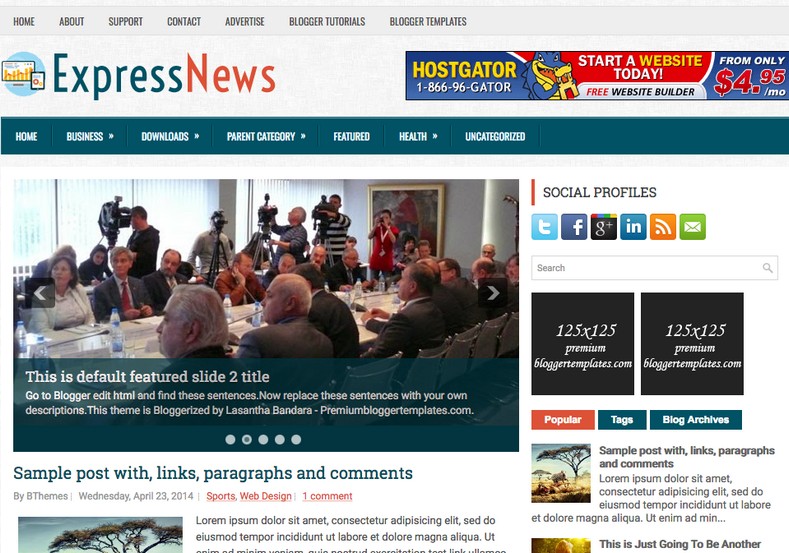This is a screen capture of the homepage of Express News, a website designed with the domain name prominently displayed in blue and red text—'Express' in blue and 'News' in red—on the top left corner. Next to this logo is an advertisement for HostGator, featuring a cartoon alligator mascot, which appears to be looking at a web page or newspaper. The ad invites visitors to "start a website today" with a "free website builder" and boasts a starting price of $4.95 per month.

Above the logo, a navigation bar includes icons for Home, About, Support, Contact, Advertise, Blogger Tutorials, and Blogger Templates, offering easy access to various sections of the site. Below the HostGator advertisement, another navigation bar features options like Home, Business, Downloads, Parent Category, Featured, Health, and Uncategorized within a blue border.

Central to the page is an image that seems to depict a business meeting or a press event, accompanied by a clickable link titled "Default Featured, Slide 2 Title" which likely allows users to read more about the featured topic.

On the far right of the screen, there are social media icons for Twitter, Facebook, Google Plus, and LinkedIn, providing quick links to the website's social media profiles. Beneath these icons is a search box for users to find specific content on the site. Toward the lower part of the page, additional headlines and images for more articles can be seen, implying a variety of news stories are available for browsing.